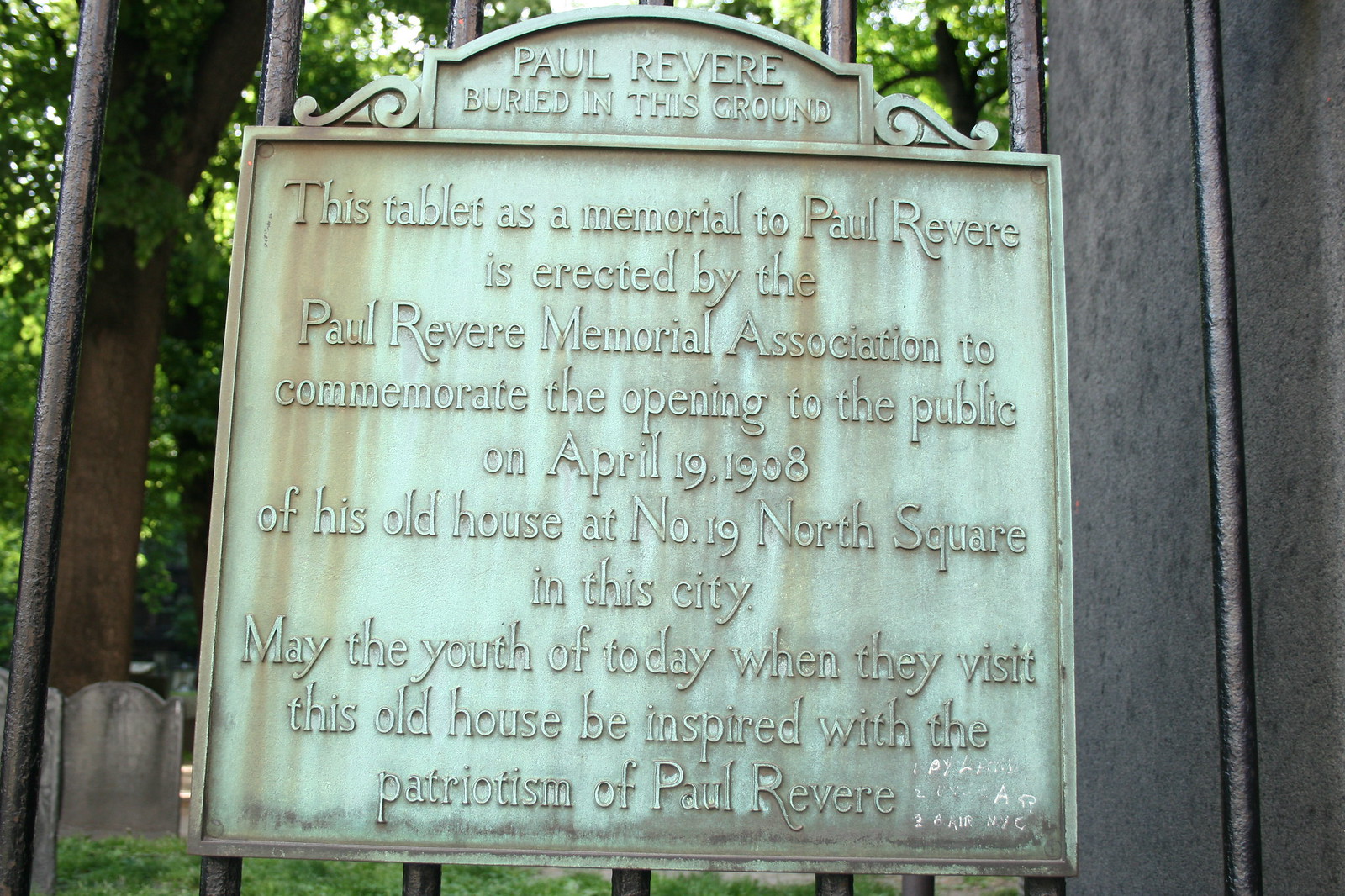The image depicts a worn, light green, metallic plaque affixed to the vertical bars of a cemetery gate. The plaque is square and shows signs of age, with patches of red rust particularly concentrated on the left and middle right sides. The inscription on the plaque reads, "Paul Revere buried in this ground." Below it, a commemorative text explains that the Paul Revere Memorial Association erected the plaque to mark the public opening of Paul Revere's old house at 19 North Square on April 19, 1908, hoping to inspire modern youth with Revere's patriotism. In the background, partially obscured by the gate and plaque, are grayish headstones and the base of a tree with numerous branches covered in leaves, indicating the setting is indeed within a cemetery.